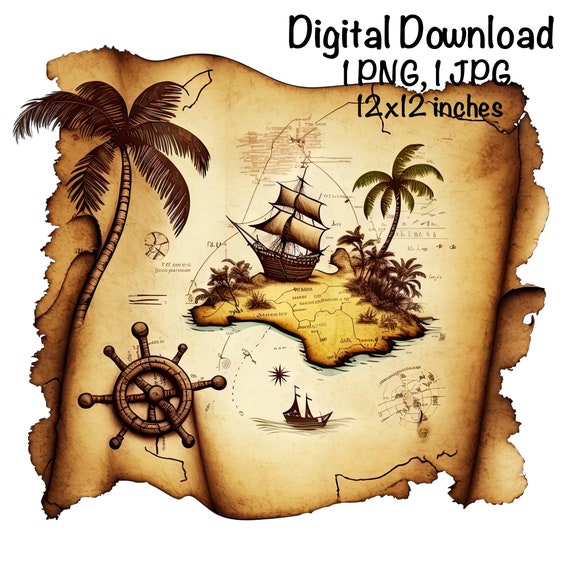This digital downloadable PNG image (also available in JPG format) measures 12 by 12 inches and features a detailed, vintage-inspired treasure map. The map, rendered in a brown, tannish color, evokes the feeling of an aged parchment guiding the viewer to hidden treasure. Prominently, on the left-hand side, a tall palm tree stands as a significant landmark. The map also intricately illustrates an old pirate ship's wooden helm, complete with thick wooden spikes serving as handle grips. Additionally, there is a marked spot indicating the presence of a boat, with another boat depicted navigating through the surrounding waters. Together, these elements create a richly detailed and immersive scene of a classic treasure hunt.